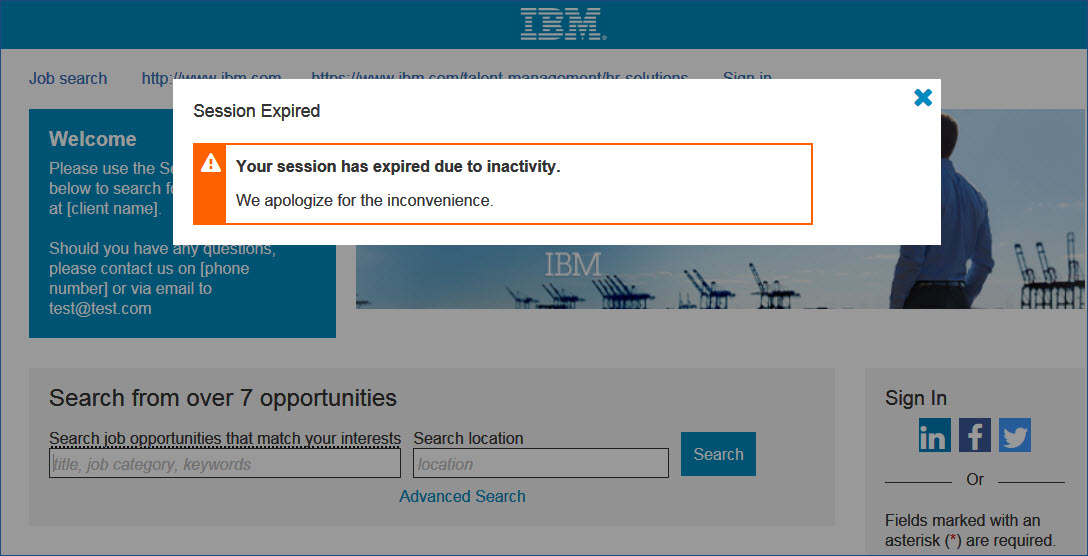In this image, a pop-up message prominently appears in the center of the screen. The pop-up message has a white background with black text, stating "Session Expired." Beneath this message, there is an orange box with the text, "Your session has expired due to inactivity. We apologize for the inconvenience." The pop-up is partially obscuring the web page behind it, which appears to be related to IBM.

At the top of the screen, a blue header bar displays the IBM logo. On the far left, the page features a navigation option labeled "Job Search." To the right of the navigation, a blue box with the text "Welcome" is partially visible. This suggests that the web page may be an IBM job or hiring portal.

Further down beneath the pop-up, we can see text indicating "search from over seven opportunities." There is also a search bar intended for users to find job opportunities that match their interests, with fields for job titles, categories, keywords, and search locations. To the right of these fields, a blue button is available for users to click and perform their job search. The overall layout and design imply that the website is focused on facilitating job searches and applications within the IBM company.